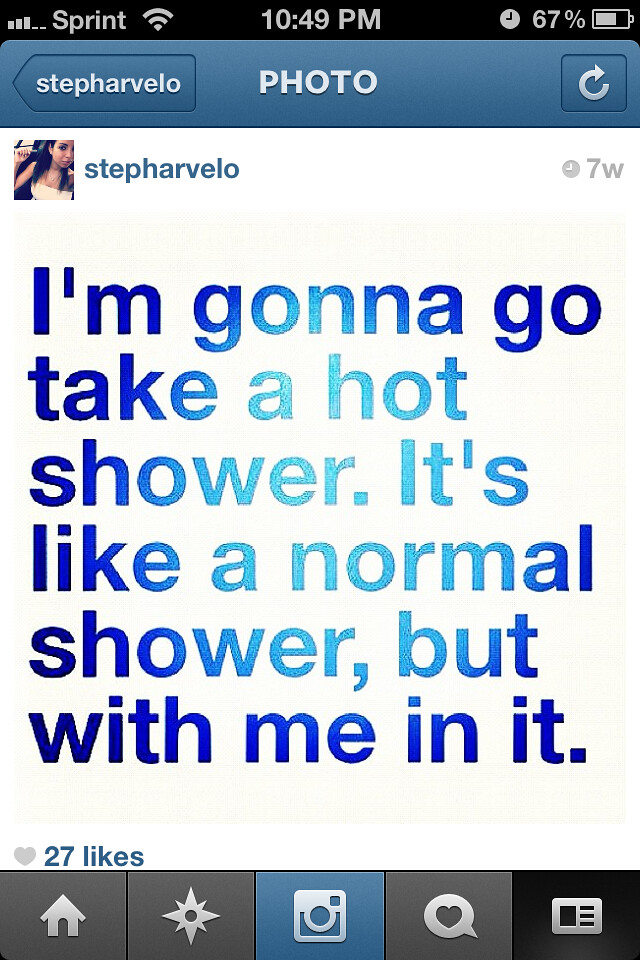This is a smartphone screenshot capturing an Instagram post from the user Stefarvelo. At the very top of the screen, the status bar shows the time as 10:59 PM, with Sprint as the carrier, a Wi-Fi icon, and the battery at 67%. Below this, in a blue tab, it says "Stefarvelo," followed by "photo" in white font. The main content shows a small square image of a woman, featuring just her torso and head, labeled "Stefarvelo." Under the image, there is a blue ombre text box stating, "I'm gonna go take a hot shower, it's like a normal shower but with me in it." This post, made seven weeks ago, has received 27 likes, indicated by a small heart icon. At the bottom of the screenshot, there is a row of icons for navigation: a home symbol, a star, an Instagram camera, a text bubble with a heart, and a news icon.